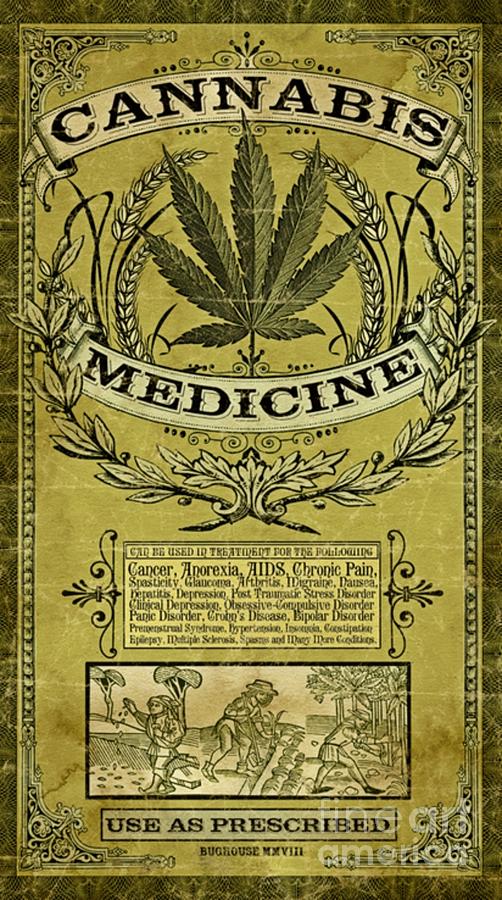The image resembles an 1800s-style rectangular poster with a predominantly yellowish-green hue and a darker green border. At the top of the poster, a white, arched banner displays the word "CANNABIS" in bold black letters. Beneath this, a prominent green cannabis leaf with seven serrated blades is depicted, surrounded by decorative arches resembling wheat. Underneath the leaf, the word "MEDICINE" is printed in an upward arched serif-style black font, and a laurel leaf design sits below it. The poster contains multiple sections, including a detailed paragraph listing various medical conditions treated by cannabis, such as cancer, anorexia, AIDS, chronic pain, spasticity, glaucoma, arthritis, migraine, nausea, hepatitis, depression, post-traumatic stress disorder, OCD, panic disorder, Crohn's disease, bipolar disorder, premenstrual syndrome, hypertension, constipation, epilepsy, multiple sclerosis, and spasms. The bottom section features rectangular images, with text and illustrations, including people possibly harvesting cannabis, and a final note stating, "USE AS PRESCRIBED" in all caps.